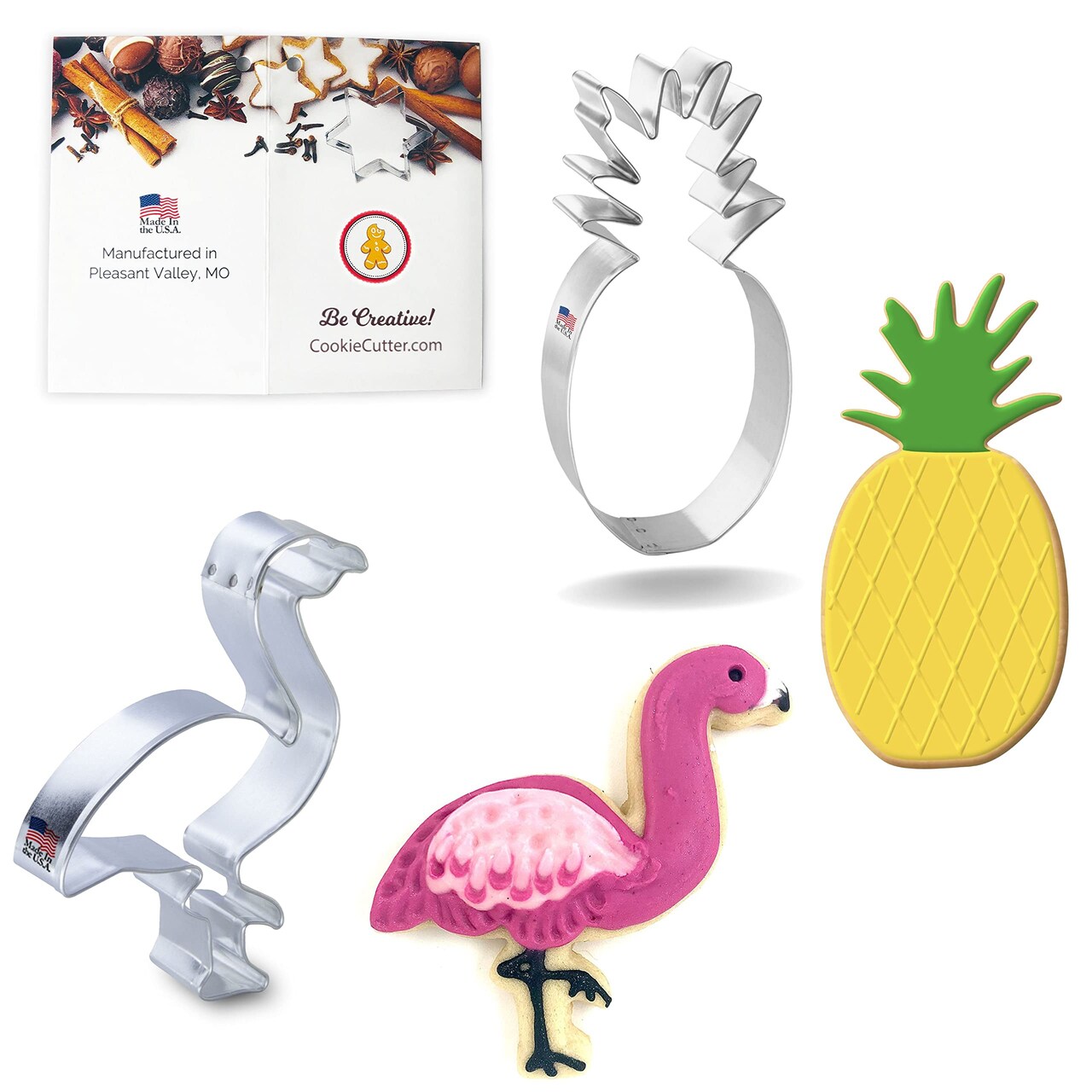The photograph features an assortment of cookie cutters and their corresponding decorated cookies, arranged on a clean white background. In the top left corner, there is a landscape-oriented brochure that is vertically folded. The left side of the brochure bears an American flag and text stating "Manufactured in Pleasant Valley, MO," while the right side displays a red circle logo with a yellow gingerbread man and the slogan "Be Creative!" above the website "cookiecutter.com." Above the brochure, various items like cinnamon sticks tied with twine, walnuts, and star-shaped cookie cutters in silver, bronze, and gold are displayed.

To the right of the brochure, a silver pineapple-shaped cookie cutter is shown with an American flag on its left side. Next to it lies a pineapple cookie, adorned with yellow icing featuring crisscross patterns and a green top.

On the left side of the image, a silver flamingo-shaped cookie cutter, also marked with an American flag at the tail, is placed. Next to it is a pink flamingo cookie with detailed icing, depicting its black legs, a tiny beady eye, and a white and black beak.

Overall, the image appears to be an advertisement for the cookie cutters, showcasing both the tools and the decorative potential of the cookies they produce.